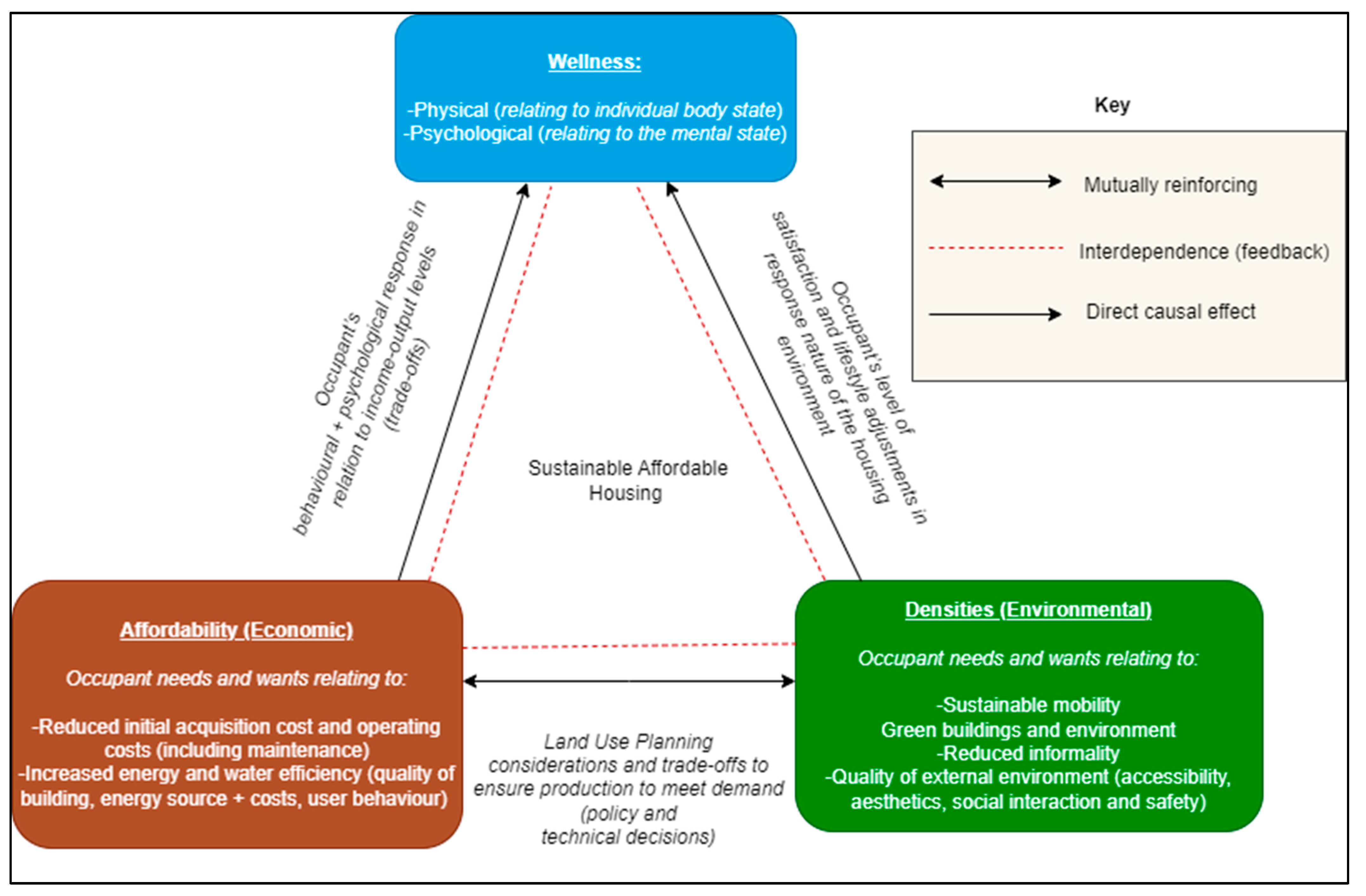This detailed diagram is composed of three interconnected squares forming a triangular relationship, and it centers around the concept of "Sustainable, Affordable Housing," prominently displayed at the triangle's core. At the triangle's apex is a blue square labeled "Wellness," which emphasizes both physical and psychological well-being. This blue square is linked to the two bottom squares via directional arrows, creating a mutual relationship among the components.

The bottom left square is red and focuses on "Affordability, Economic," which includes factors such as economic affordability and income-related trade-offs. On the bottom right is a green square labeled "Densities, Environmental," highlighting elements like sustainable mobility, green buildings, and reduced informality.

The diagram also features detailed descriptions of each section. On one side of the triangle, there's a note about occupants' behavioral and psychological responses in relation to their income output levels and trade-offs. The other side mentions occupants' levels of satisfaction and lifestyle adjustments in response to the nature of the housing environment.

Additionally, there is a key on the right side of the diagram, which clarifies how these components interrelate—whether they work mutually, independently, or in a cause-effect manner. This comprehensive chart effectively communicates the interconnected factors essential for sustainable and affordable housing, making it suitable for presentation at a board meeting or similar professional setting.